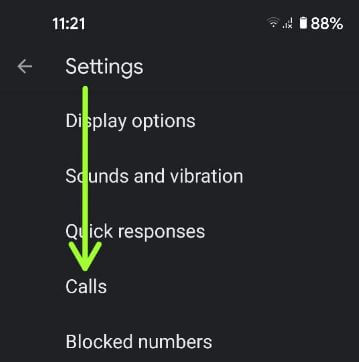This is an amended screenshot of a smartphone settings page. The time "11:21" is displayed at the top left corner, and on the right side, there are status icons for WiFi, mobile data, and the battery, which is at 88%. The screen has a dark background. The word "Settings" is prominently displayed at the top of the page, below which there is a list of options: "Display options," "Sounds and vibration," "Quick responses," "Calls," and "Blocked numbers." A green arrow, manually drawn on the screenshot, starts at "Settings" and passes through "Display options," "Sounds and vibration," and "Quick responses," ultimately pointing to the "Calls" option. The purpose of the arrow is not explicitly mentioned, suggesting it might be part of a larger instructional guide or tutorial for altering call settings on the device.